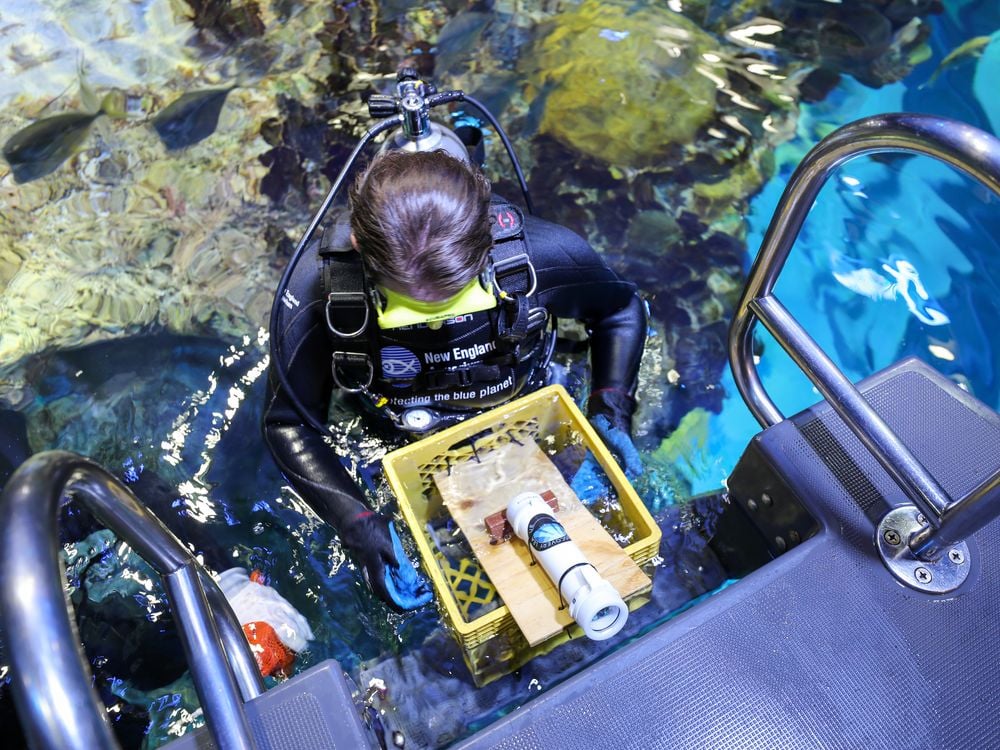From the vantage point above, the image captures a female scuba diver in full gear ascending a ladder at the back of a boat. The diver, clad in a black wetsuit with the words "New England protecting the blue planet," is holding a yellow crate filled with various tools, including a piece of wood and a tube. Her goggles are yellow, contrasting with the primarily dark coloration of her attire. Her gloves are dark with light blue accents on the palms. The water below is remarkably clear and blue, revealing a vibrant underwater scene with visible rocks, plant life, and a few fish, including one in the top left corner. Silver railings flank the gray ladder that she is using to climb out of the water.